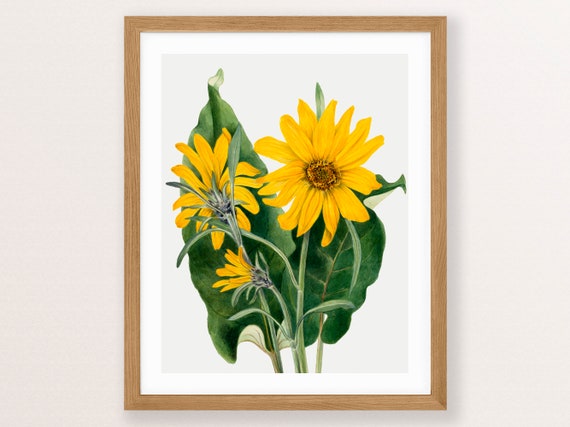The image captures a framed watercolor painting, meticulously housed in a light wooden frame with a solid white inset. This artwork, hung on an almost white wall, presents a delicate illustration of three yellow flowers, each with detailed yellow petals. The top right flower is facing forward in full bloom, while the left one is oriented away. Below these two, a smaller flower is emerging from its bulb. Behind them, large green leaves and thick green stems rise from the bottom, creating a vibrant backdrop against the painting’s white background.